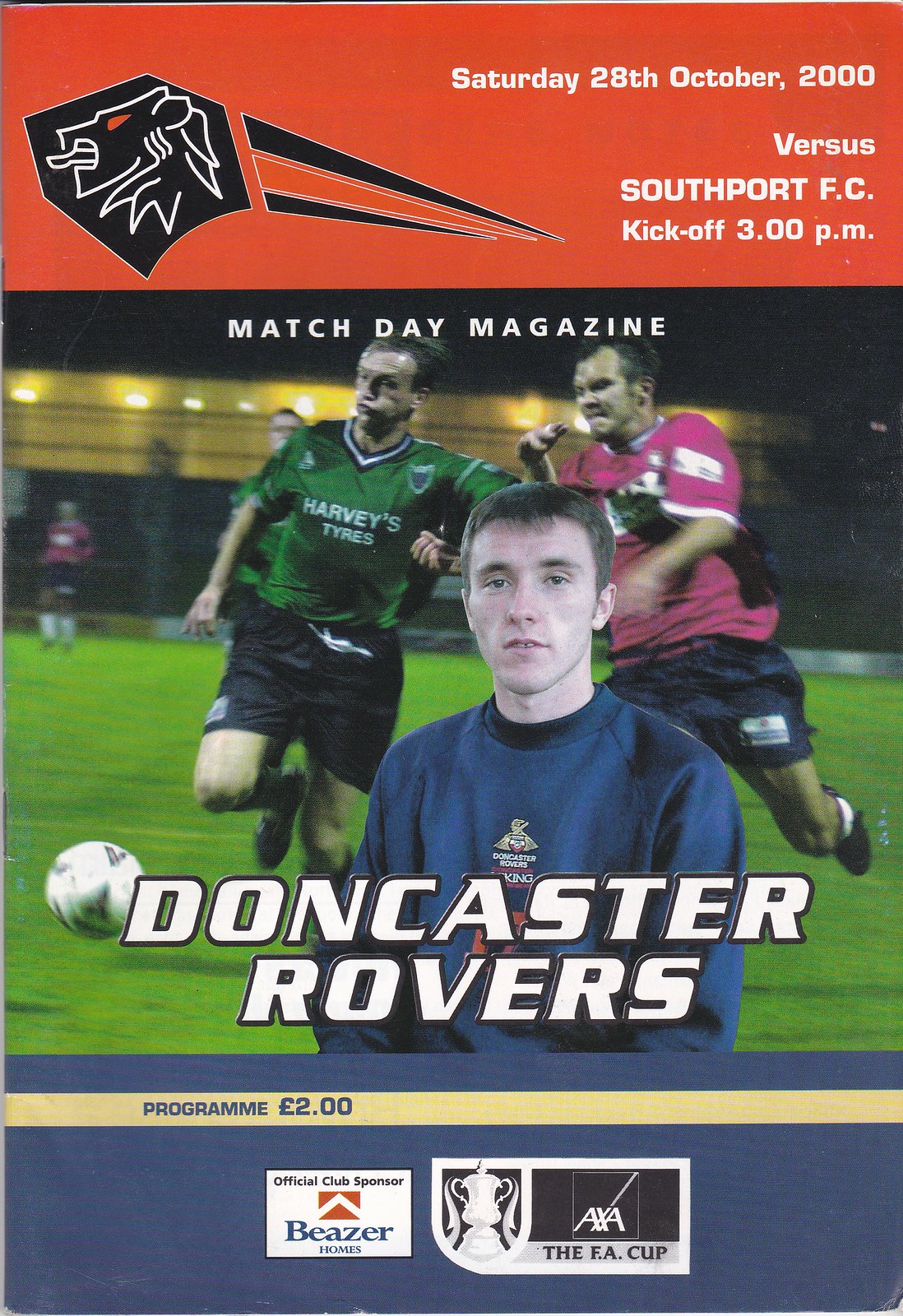The image is the cover of a sports program, advertising a sporting event. At the top, a red banner with white font announces "Saturday, 28th October 2000 versus Southport F.C. kickoff 3 p.m." Beneath this red area, the header reads "Match Day Magazine" with "Doncaster Rovers" prominently displayed in large white font. The main visual features three men. One man stands in the foreground, facing the camera, wearing a blue long-sleeve shirt with "Dorchester Rovers" written on it. Behind him, two men, seemingly engaged in a soccer match, are captured mid-action—one in a green shirt labeled "Harvey's Tries" and another in a brightly colored pink shirt. The bottom part of the cover has a blue box intersected by a yellow line, with "Program £2.00" written in blue font on the yellow stripe. Two sponsor logos, Beezer Homes and the FA Cup, are positioned beneath this section. An emblem featuring a lion with radiating lines is placed to the side, adding to the dynamic design of the program cover.